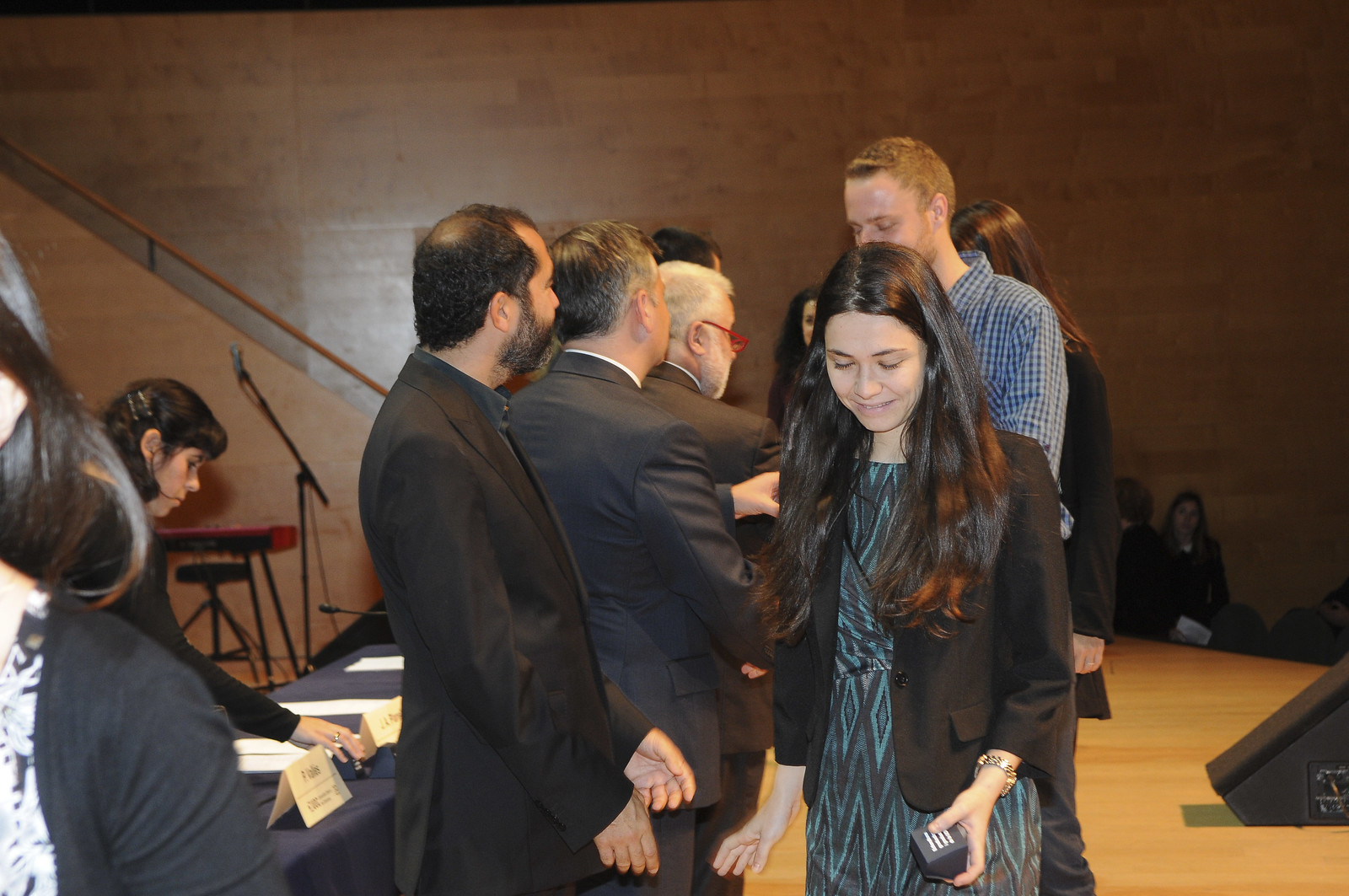The photograph captures a scene on an elevated stage where people are lining up, seemingly for a ceremony or event. The background features a paneled wall made of polished, light brown wood, contributing to the warm, inviting atmosphere. On the left side of the image, a set of stairs with a brown railing leads up to the stage. The stage floor is made of light-colored wood, and in the background, a lower area with more people is visible, adding depth to the setting.

A long table draped with a black tablecloth runs along the left side of the stage. On this table, multiple white name cards and papers are neatly placed, and a woman with long, dark hair is in the process of arranging something on it. The focus of the image is on a young woman, probably in her early 20s, with long dark hair, standing at the front of the line. Behind her is a man in his late 20s or early 30s with blonde hair, wearing a blue plaid shirt.

Further in the background, several older men, likely in their 40s and 50s and dressed in dark suits, are shaking hands with the people in line, possibly handing out items or congratulating them. This indicates that a formal gathering, such as a graduation or an award ceremony, is taking place, characterized by the poised interactions and well-dressed attendees.